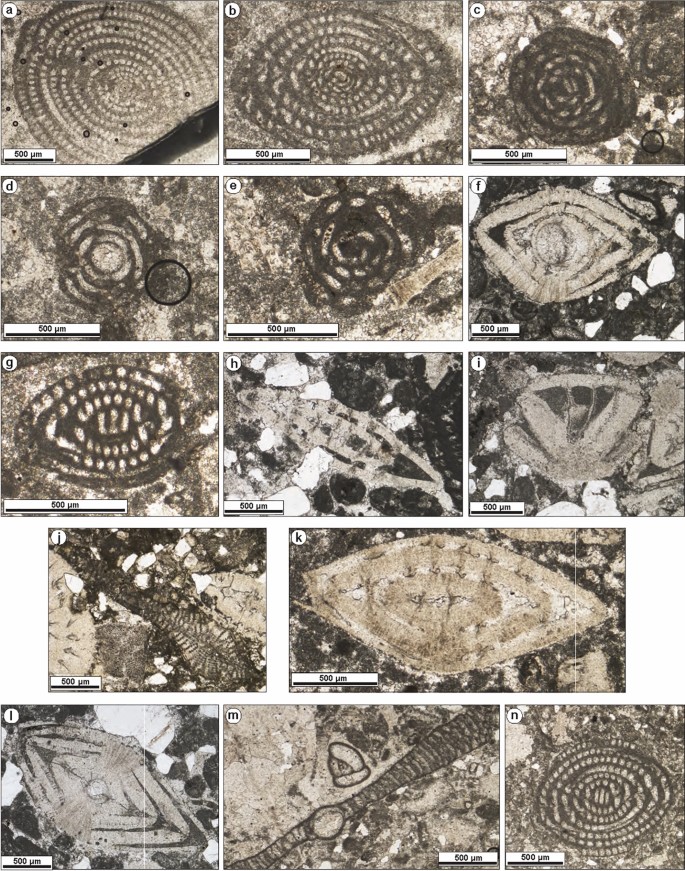The image is a compilation of 14 smaller black and white photos, each labeled in the upper right-hand corners from A through N. These images present aerial or microscopic views of various shapes and patterns on the ground, predominantly circular with some almond and oval shapes. The shapes range in color from light gray to black. Each photo is annotated in the lower left-hand corner with '500YM' or '500 micrometers,' though the exact label isn't entirely clear. The layout appears to follow a scientific slide format: the top row consists of images labeled A, B, and C, showcasing mostly elliptical shapes; the second row contains D, E, and F with more circular forms; the third row includes G, H, and I; the fourth row features J and K, with K being slightly more rectangular or triangular; and the final row displays images labeled L, M, and N, showing various scientific representations. Notably, three of the images have a black circle drawn within them. The images exhibit intricate details, making it difficult to discern whether they are satellite photos from a high altitude or microscopic views of tiny objects.